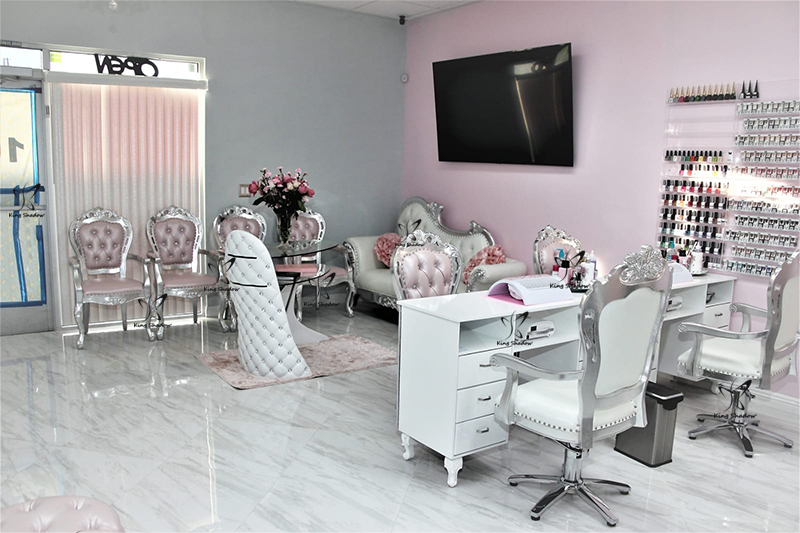The photograph captures a luxurious nail salon setting with an elegant and thoughtfully designed decor. The waiting area features white and pink high-end leather couches and chairs, each accented with silver linings. In the center, there's a table adorned with pink flowers in a vase. A large flat-screen TV is mounted on the back wall, accompanied by an "open" sign above white blinds, beside a window.

The flooring throughout the salon is a sleek white and gray marble. To the right, a display case exhibits an array of colorful nail polishes, beside which are two white leather desks, each with matching silver-bordered chairs for the technicians. In between these chairs rests a silver garbage can.

The walls on the right side are lavender, while those on the left side are a lighter gray. In addition to the lavish chairs, there are soft pink curtains near the front door and a light blue couch positioned in the background. A pink carpet adds a touch of warmth and contrasts subtly with the marble floor.